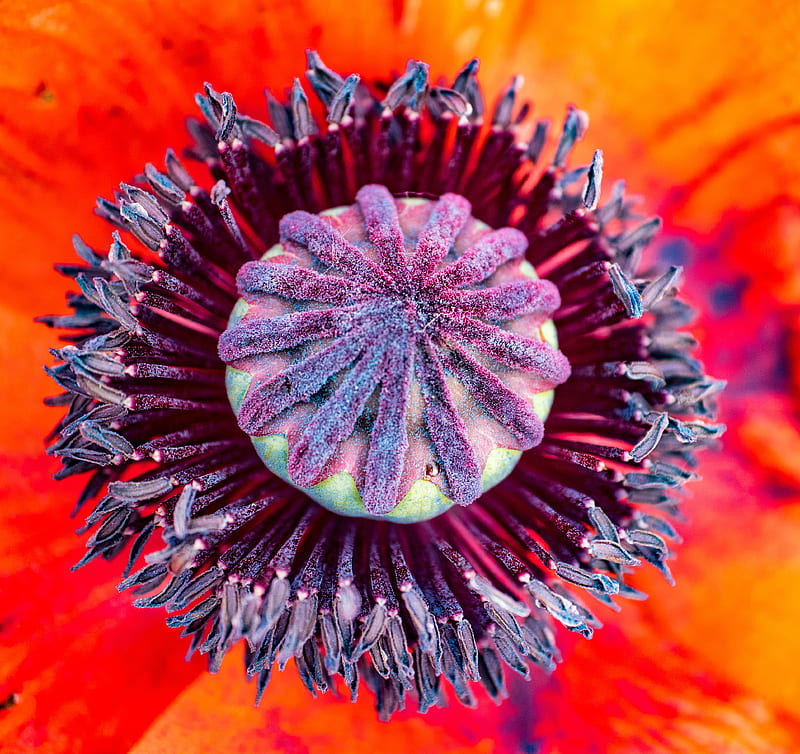This detailed macro shot captures the mesmerizing center of a flower in full bloom, likely a poppy, showcasing a vivid display of colors and intricate details. The petals extend outward with stunning shades of orange, red, and yellow, creating a molten lava-like effect. At the heart of the flower is a green, circular structure adorned with bluish-purple florets, surrounded by tiny, pollen-covered filaments. The central part of the flower features a dense, textured green nugget encircled by fur-like rays that resemble a clock dial, adding to the vibrant complexity. The brilliant interplay of greens, blues, maroons, and purples against the bright, burnt orange and yellow background makes the image not just a visual feast but almost reminiscent of a piece of vivid, colorful art.